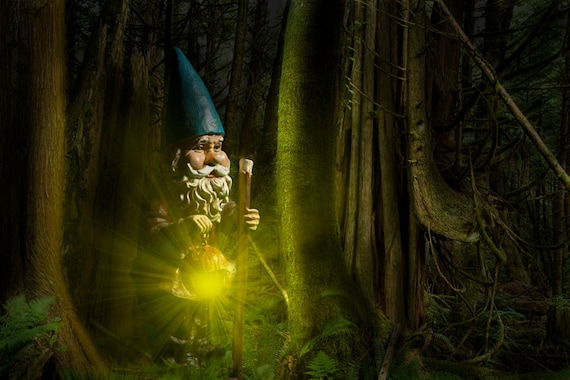The image depicts a digitally generated, fantasy-themed scene set in a dark forest with dense green foliage, tree trunks, and various plants. At the center, there is a garden gnome-like figure, which has long, wavy white beard and mustache and wears a blue conical hat. The gnome is dressed in a robe-like garment and appears worried, as indicated by its serious facial expression. It is nighttime, evident from the dark sky and the shadowy trees surrounding the figure. The gnome is holding a spherical lantern emitting an eerie green light in one hand, and a wooden cane in the other, using the lantern to navigate through the forest.